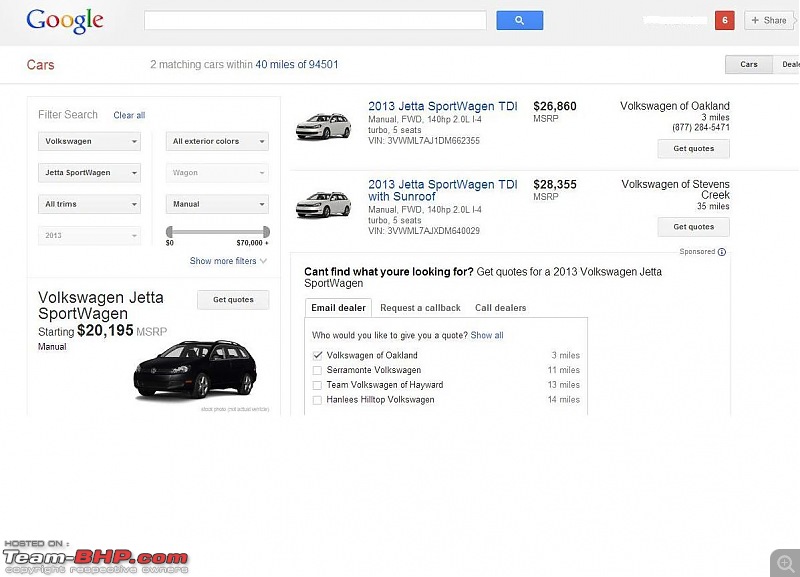The image depicts a search results page with Google branding in the top left corner. Adjacent to the Google logo is a long, empty search bar in white, followed by a small blue rectangle featuring a magnifying glass icon. To the right of the search bar, there is a red square with the number '6' inside. Beneath the Google logo, aligned to the left, is the word "cars." To the right, it states, "two matching cars within 40 miles of 94501."

Further down the page, there are two car listings. On the left, an image of a silver 2013 Jetta Sport Wagon is shown with a price tag of $26,860 MSRP. There is a clickable area labeled "Get Quotes." To the right of this, the second listing also features a 2013 Jetta Sport Wagon, but with a sunroof, priced at $28,355 MSRP. This vehicle is available at Volkswagen of Stevens Creek and includes a clickable "Get Quotes" option.

In the lower left corner of the page, another Volkswagen Jetta Sport Wagon is displayed, this one starting at $20,195 MSRP and shown in black. The webpage is hosted on team-BHP.com, which is prominently displayed in red capital letters in the bottom left corner.